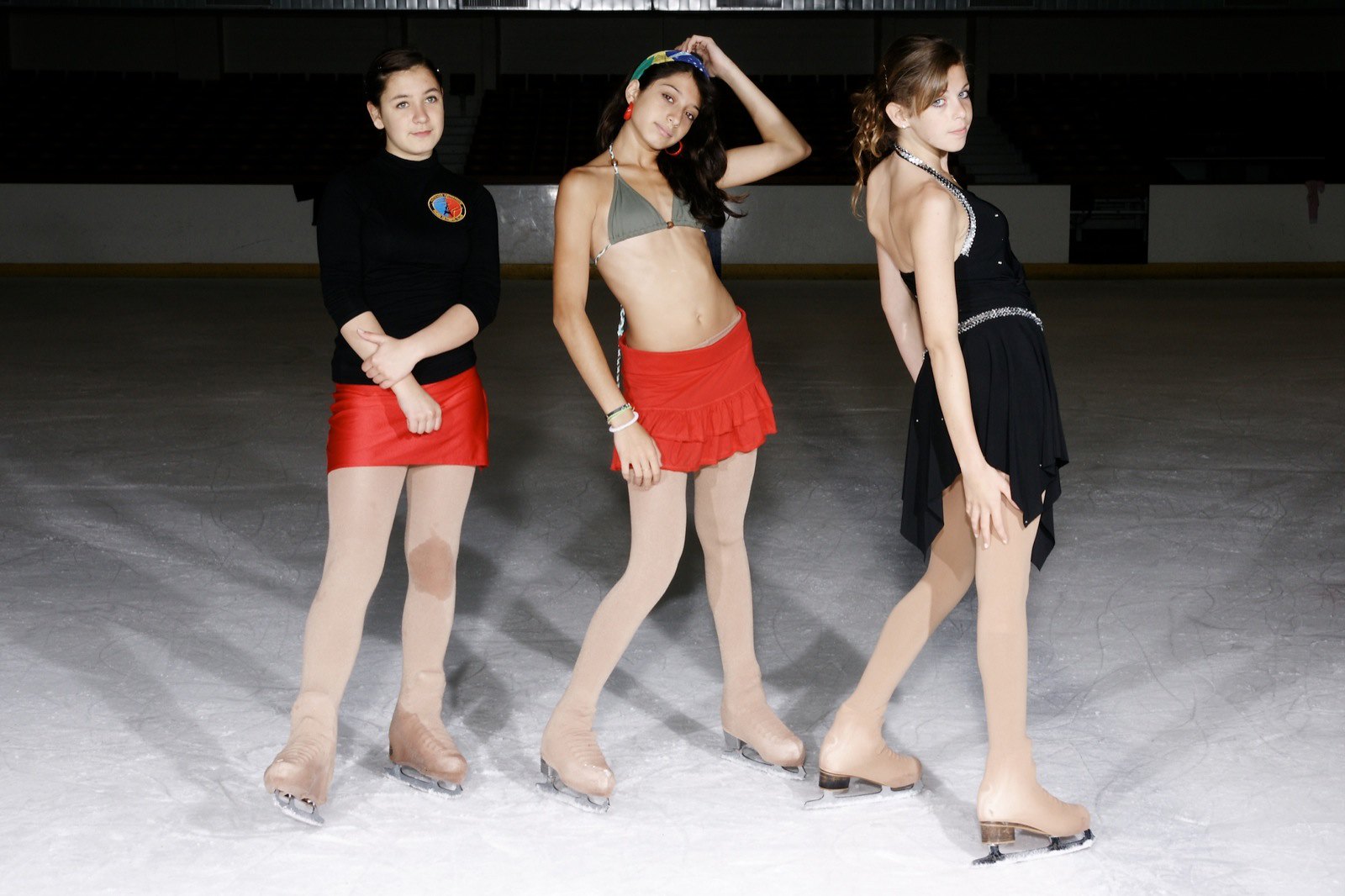In this detailed photograph, we see three young female figure skaters posing on a white ice rink, set against white boards. The skater on the left is wearing a red skirt paired with a black top adorned with a red and blue circular logo. She has her dark hair pulled back and appears shy, holding one arm with the other. The middle skater, showcasing an adventurous spirit, sports a gray bikini top and a short red skirt with flippy details. Her long, curly dark hair is held back by a colorful green and blue headband, and she accessorizes with red hoop earrings. Her pose has one arm raised above her head and the other to the side, with her head slightly slanted. The skater on the right is dressed in a black, sequined halter-style ice skating costume, trimmed with silver sequins around her waist and neck. She has her hair pulled back into a curly ponytail, with the front straightened, and poses with her back to the camera, looking over her shoulder. All three skaters are wearing light brown nylons that match their brown ice skates, giving a seamless aesthetic to their elegant presence on the ice.